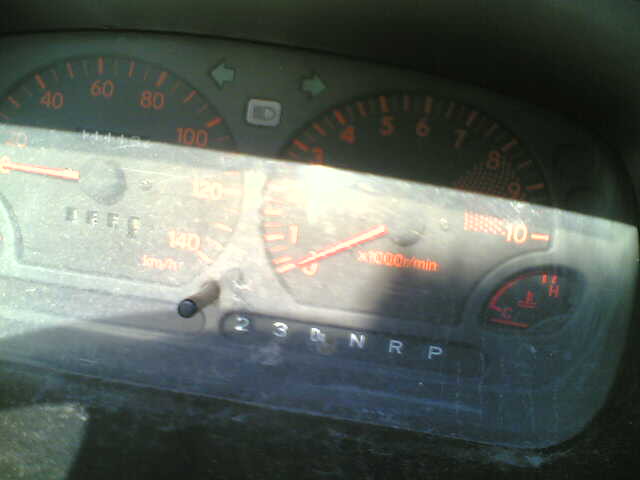This photograph depicts a vintage car's dashboard, focusing on the speedometer. The speedometer dial, though somewhat blurry, showcases various essential gauges. On the left and right, there are signal indicators for turn signals. A temperature gauge, ranging from cold to hot, can also be seen. It's challenging to decipher whether the tachometer reads 3 or 1000 RPM due to the blurry quality of the image.

All the gauges are housed behind a murky layer of glass or plastic, urgently needing cleaning, perhaps with Windex. The sunlight partially illuminates the dashboard, with some light obstructed by the window frame, resulting in a mix of bright and shadowed areas.

Additionally, the gear selector display is visible, indicating "23DNRP" for the Park, Reverse, Neutral, and Drive positions, alongside the numbers one and two. The overall setup suggests this is an older model vehicle, exuding a nostalgic charm despite the dirty lens and harsh lighting conditions.